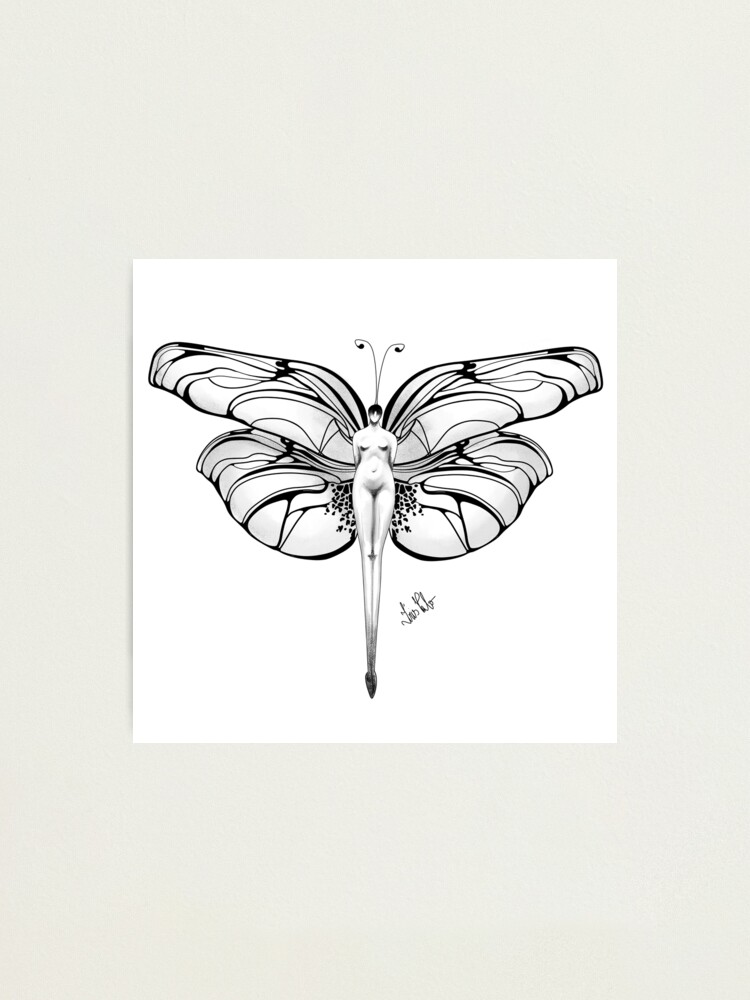This image showcases a black and white drawing set against a pale gray background. The artwork, about 8x8 inches in size, depicts a fanciful butterfly with intricate wing details, including veins and segments. The butterfly’s body, however, is uniquely replaced by the figure of a nude woman. Her arms are either hidden behind her or absent, reminiscent of the Venus de Milo statue. The woman's anatomy, including her breasts, pubis, belly, and exceptionally long legs, tapers elegantly into the butterfly's tail, resembling a swallowtail butterfly. She also features two antennae extending from her head. The drawing is signed by the artist in the bottom right corner, with the last name starting with a 'P,' though the full signature remains indistinguishable. The image is simplistic yet detailed, with the butterfly and woman rendered in a purely monochromatic scheme and centered on the white paper.